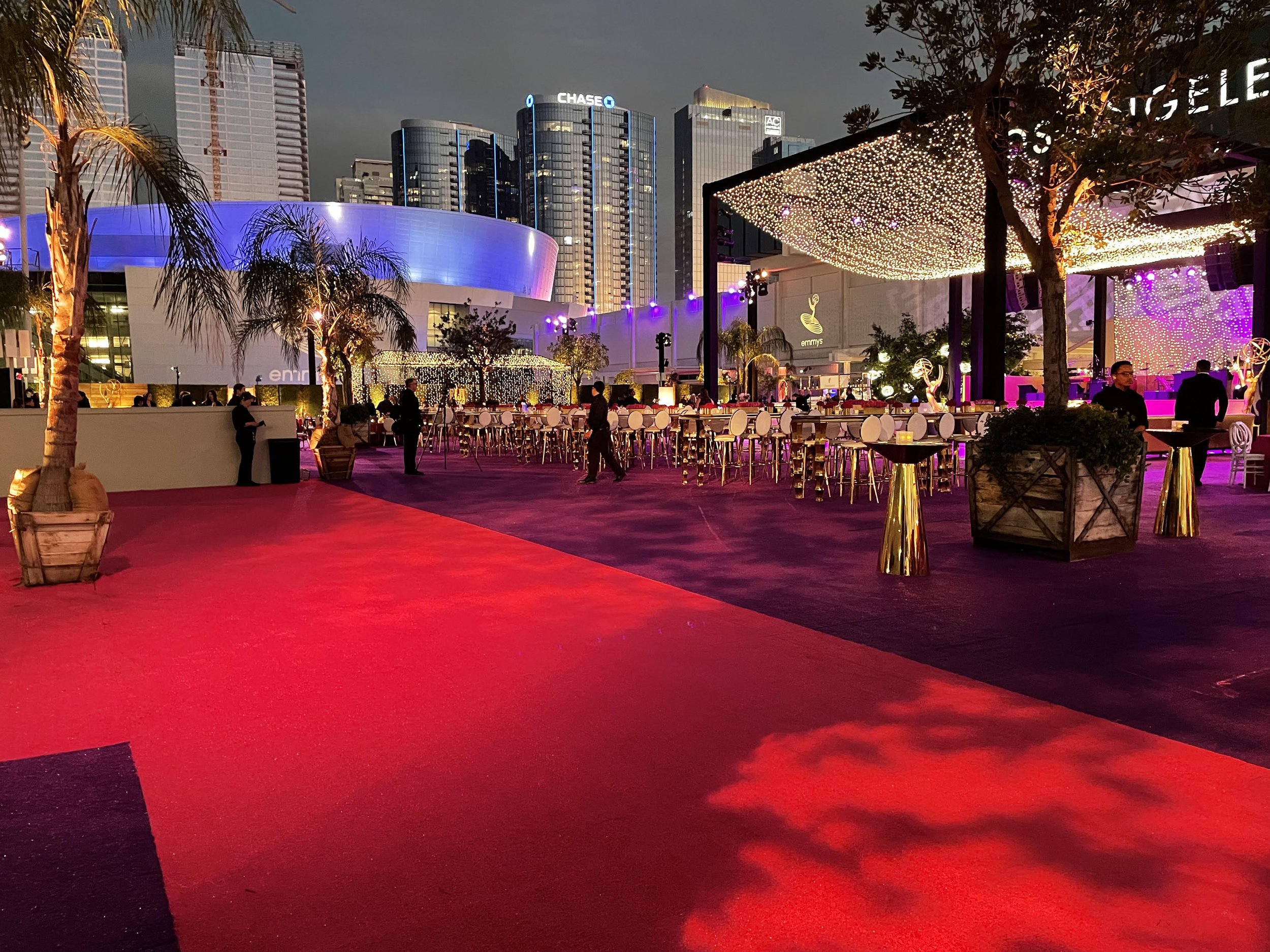In a captivating outdoor nighttime setting within a bustling city, this photographic image captures the vibrancy of a luxurious urban event, possibly a restaurant or a nighttime party. The foreground prominently features a striking red carpet that blends seamlessly into a deep purple one, bordered by numerous high chairs and tables suggestive of an upscale dining or social area. A lush array of palm trees in baskets adds a tropical flair, subtly swaying under the ambient city lights.

In this lavish scene, a man dressed entirely in black walks away while another stands, exuding an air of sophistication. Although the area seems sparsely populated, a closer look reveals more individuals: a woman sits to the bottom right, in front of a tree, with a man leaning against a nearby wall behind her, both clothed in formal attire.

The backdrop is a stunning display of towering skyscrapers with sleek gray and steel facades, epitomizing modern urban architecture. One skyscraper proudly bears the Chase logo, while another building on the top right corner features the illuminated text "Los Angeles." Moreover, a building in the left-hand corner is distinguished by its curved purple roof, enhancing the venue's visual allure. Festive, stringed lights add to the evening's enchantment, casting a soft glow over this elegant cityscape.